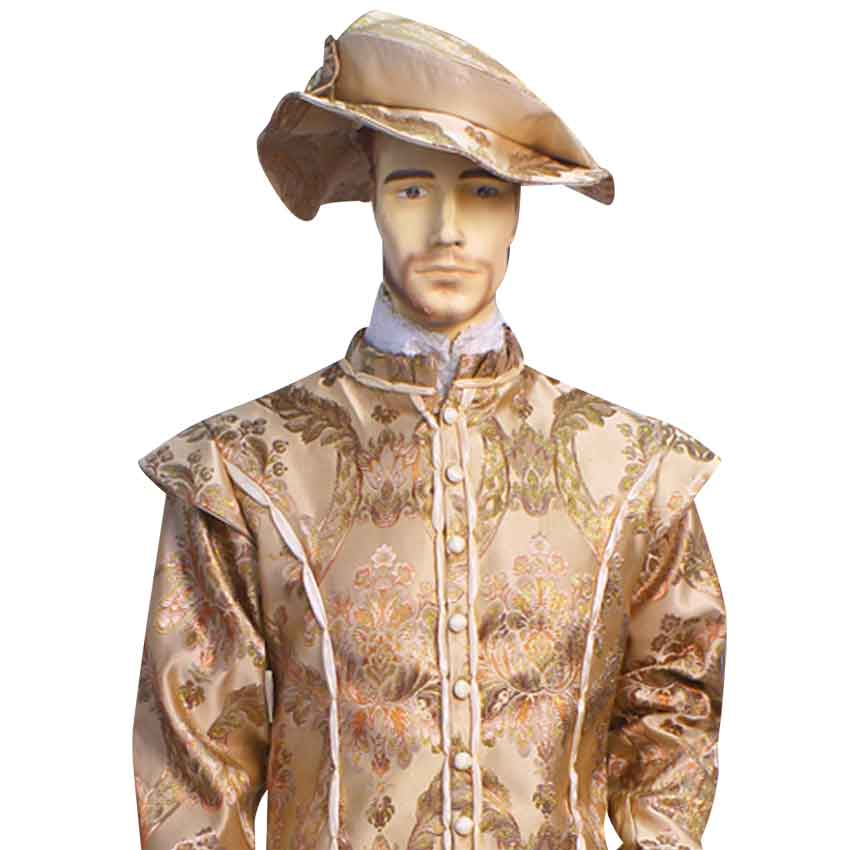The image depicts a lifelike male mannequin wearing an elaborate, Renaissance-inspired outfit. The mannequin sports a well-trimmed goatee and dark eyes, accentuating its lifelike features. The attire includes a visually striking, silky, golden brown hat adorned with intricate floral patterns, slightly tilted to one side. This hat complements a matching, elaborately embroidered jacket or coat, also golden brown, with a floral design that spans its entirety. The coat is fastened with a row of large, circular white buttons that resemble pearls. Beneath the coat, a white undershirt with ruffled details at the neck is visible, adding to the historical feel of the ensemble. The shoulders of the main garment are slightly padded, creating a distinguished silhouette. The overall outfit, rich in detail and reflective of ancient craftsmanship, evokes the attire of a guard or noble from centuries past.